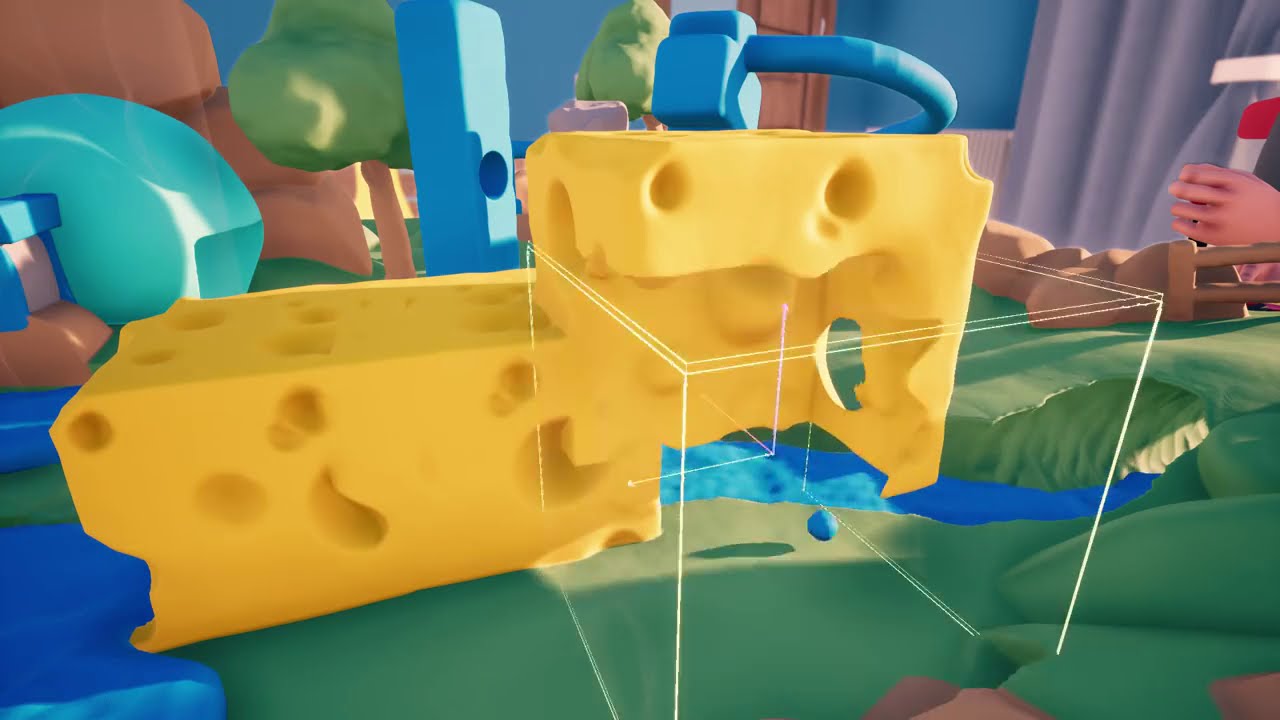The screenshot from this video game presents a meticulously crafted 3D rendering, featuring a vibrantly detailed landscape. In the foreground, two large blocks of Swiss cheese, characterized by their signature holes, rest upon a lush green ground. Below one of these cheeses is a white outline of a cube, adding an intriguing geometric element. Surrounding this scene, a river with vivid blue water meanders, contrasting beautifully with the greenery. Beyond the river, a variety of colorful objects can be seen, alongside several brown rocks and towering mountains. Adding to the tactile nature of the image, everything appears to be fashioned from plastic or clay, evoking a whimsical, toy-like quality. Additionally, a 3D-rendered hand is visible on the right side of the frame, holding a white stick with a red tip, enhancing the interactive feel of the scene. In the backdrop, green hills dotted with trees and large stone cliffs create a picturesque setting, while a rustic brown fence provides a charming final touch to this richly detailed virtual world.